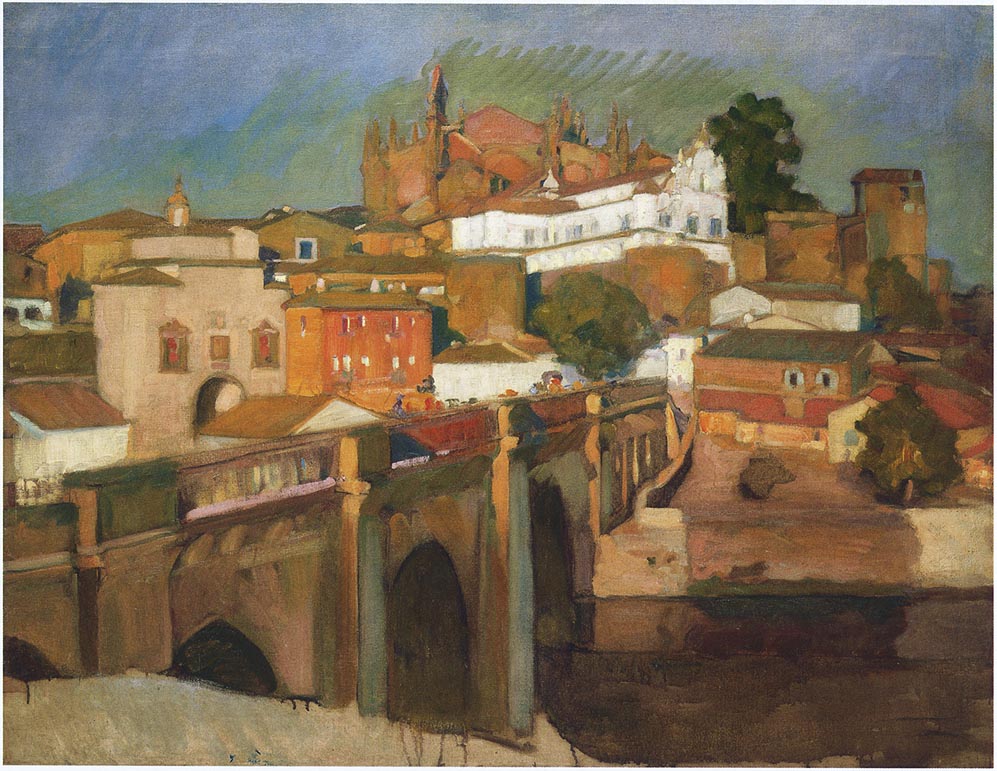This detailed painting depicts a quaint village nestled on a hillside. In the bottom left corner, a winding hillside leads to a long, brownish bridge that stretches towards the village. On the bridge, small dots of color represent numerous people, some standing and gazing into the distance or down towards the dark, blackish river below.

The village appears to climb the hill, with buildings seemingly rising higher, although their individual heights do not change. The buildings are a mix of red, light gray, and white, the latter featuring dome roofs that stand out prominently. At the summit of the hill, a large structure resembling a castle or a church dominates the skyline, imbuing the scene with a sense of historical charm.

The painting uses somber, dark colors, with a sky that blends dark blue and green hues. Scattered throughout the scene are trees, particularly noticeable at the top right, bottom left, and far right, adding touches of natural beauty to the composition. The overall atmosphere of the painting is peaceful yet mysterious, capturing the essence of a serene village moment frozen in time.